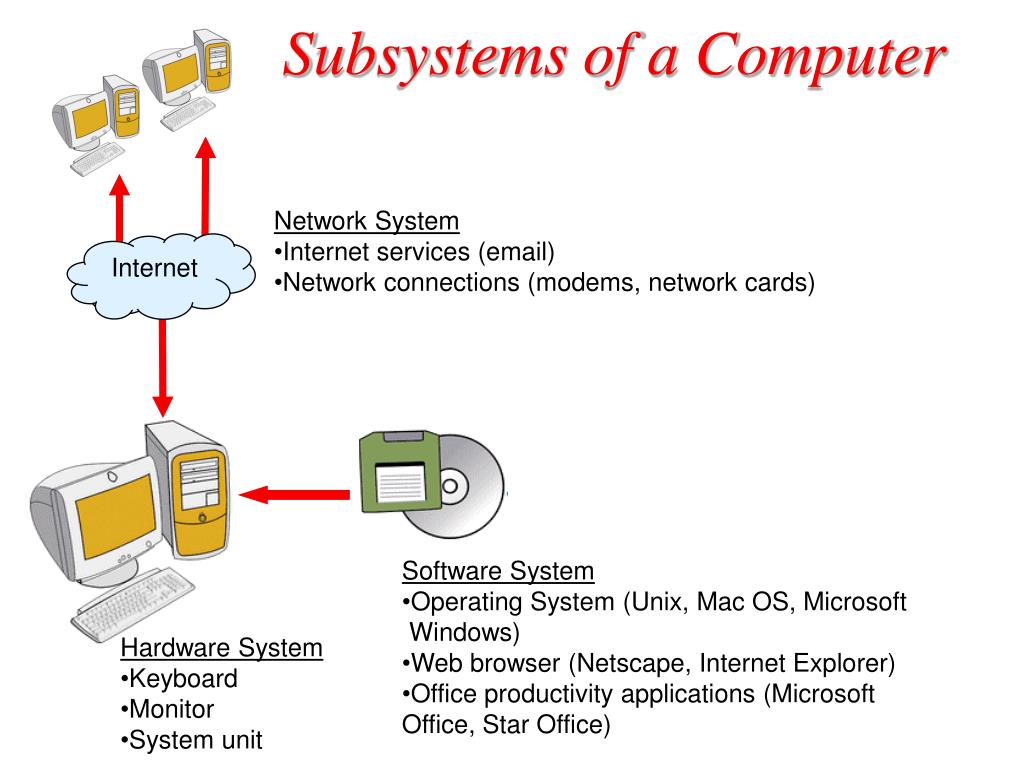The diagram titled "Subsystems of a Computer," presented in red italicized font at the top center on a white background, visually explains three main components using text and illustrative icons. In the top left corner, it features two vintage desktop computers, each with a white monitor and a yellow screen next to yellow-front computer towers. Below this, a light gray cloud labeled "internet" in black text has red arrows extending upwards to the computers and downwards to a larger computer setup below, indicating internet connectivity.

To the right of the cloud, underlined black text reads "Network System," with bullet points listing "Internet Services (email)" and "Network Connections (modems, network cards)." Adjacent to the larger computer, the section labeled "Hardware System" in underlined black text includes bullet points for "Keyboard," "Monitor," and "System Unit."

To the right of the larger computer setup, a green floppy disk and a gray CD are depicted, accompanied by underlined black text reading "Software System." This section lists operating systems (Unix, Mac OS, Microsoft Windows), web browsers (Netscape, Internet Explorer), and office productivity applications (Microsoft Office, StarOffice) as bullet points.

The diagram merges visual elements and text to provide a comprehensive overview of computer subsystems, specifically illustrating network, hardware, and software components with corresponding connections and examples.